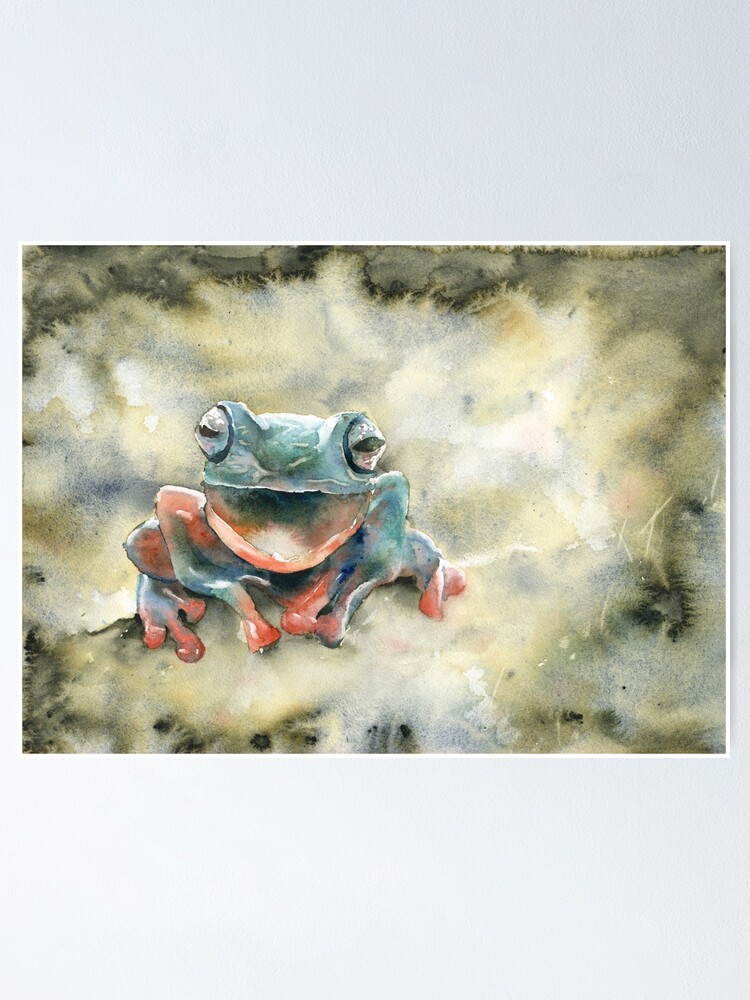This watercolor painting artfully depicts a teal-colored tree frog with distinctive bulbous, red fingers and toes, three on each hind foot. The frog features large, aquamarine bulging eyes with horizontal black slits, creating a striking focal point. Its smooth, scaleless skin is vividly illustrated, with accents of yellow and orange around its body. The frog, appearing as if staring directly at the viewer, has its mouth open wide, contributing to its lifelike yet artistically expressive portrayal. It is perched on an indistinct surface, possibly a tree branch. The background comprises a blend of muted yellows, whites, browns, and blacks, executed in a splotchy, marbled watercolor style reminiscent of stains left by spilled liquid, enhancing the overall aesthetic appeal.